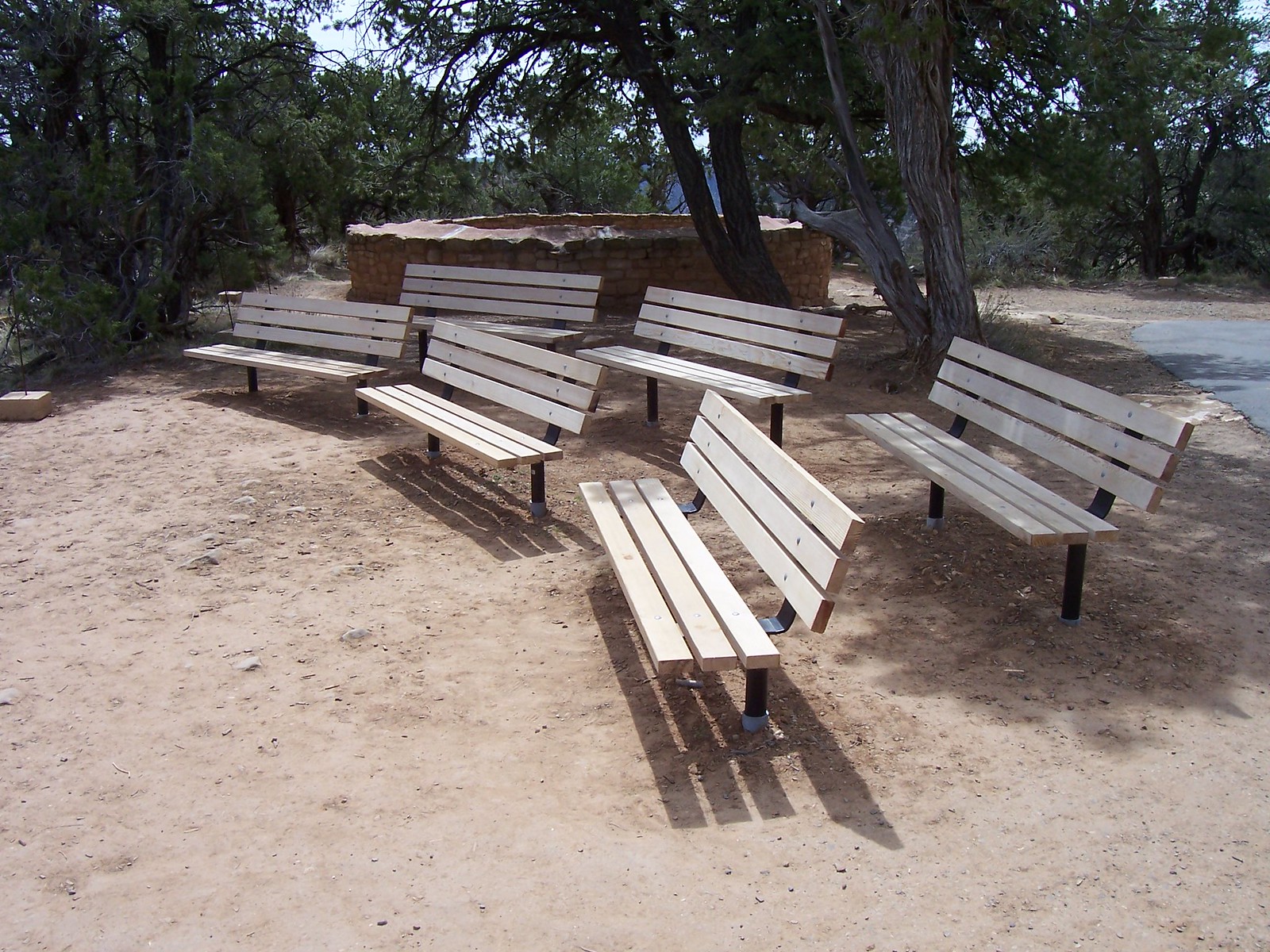The photograph captures an outdoor setting in a wooded park with flat, tan-colored dirt and no visible grass. Central to the image are six park benches, arranged in two slightly curved rows of three. Each bench is constructed from light blonde wood planks - three for the seat and three for the back - supported by sturdy black metal legs that appear cemented into the ground. The benches all face the same unseen focal point, perhaps indicative of an area designated for events or gatherings.

Behind the benches is a significant circular brick structure, reminiscent of a well or pit, open in the middle and sizeable enough to be notable. Surrounding this seating arrangement and brick feature are multiple trees, with trunks ranging in color from light brown to dark gray, and canopies full of green leaves. A gray path or road can be seen to the right of the trees, and patches of sky peek through the foliage, suggesting it is daytime. The overall scene suggests a tranquil, purposefully arranged area within a larger park.